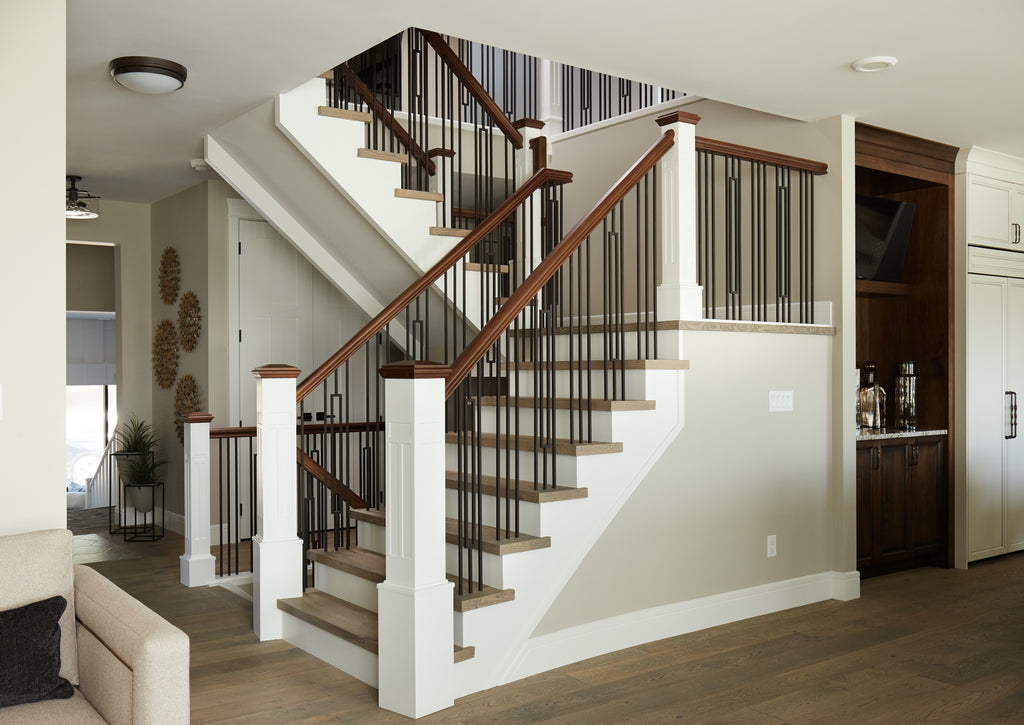The photograph captures the interior of a well-lit house featuring prominent white walls and ceilings. Centrally, a staircase commands attention with its dark brown wooden guardrails and intricate, darker metalwork balusters. The stairs begin with two white pillars on either side, ascend half a flight to a landing, then turn left before continuing upward to the next level. Additionally, a stairway to the basement is hinted at beside the main stairs. The flooring is a light brown hardwood, which extends throughout the scene.

In the lower left corner, there’s an off-white, almost light beige leather or vinyl sofa adorned with a small, dark, possibly velvet throw pillow. Just beyond the staircase, to the right, lies the kitchen area, featuring a dark wood bar with cabinets and containers, a white pantry, and more wooden cabinetry above the counter. Further details include a window with blinds and a light above it, some wall hangings, and a potted plant, all adding to the cozy ambiance of the interior.